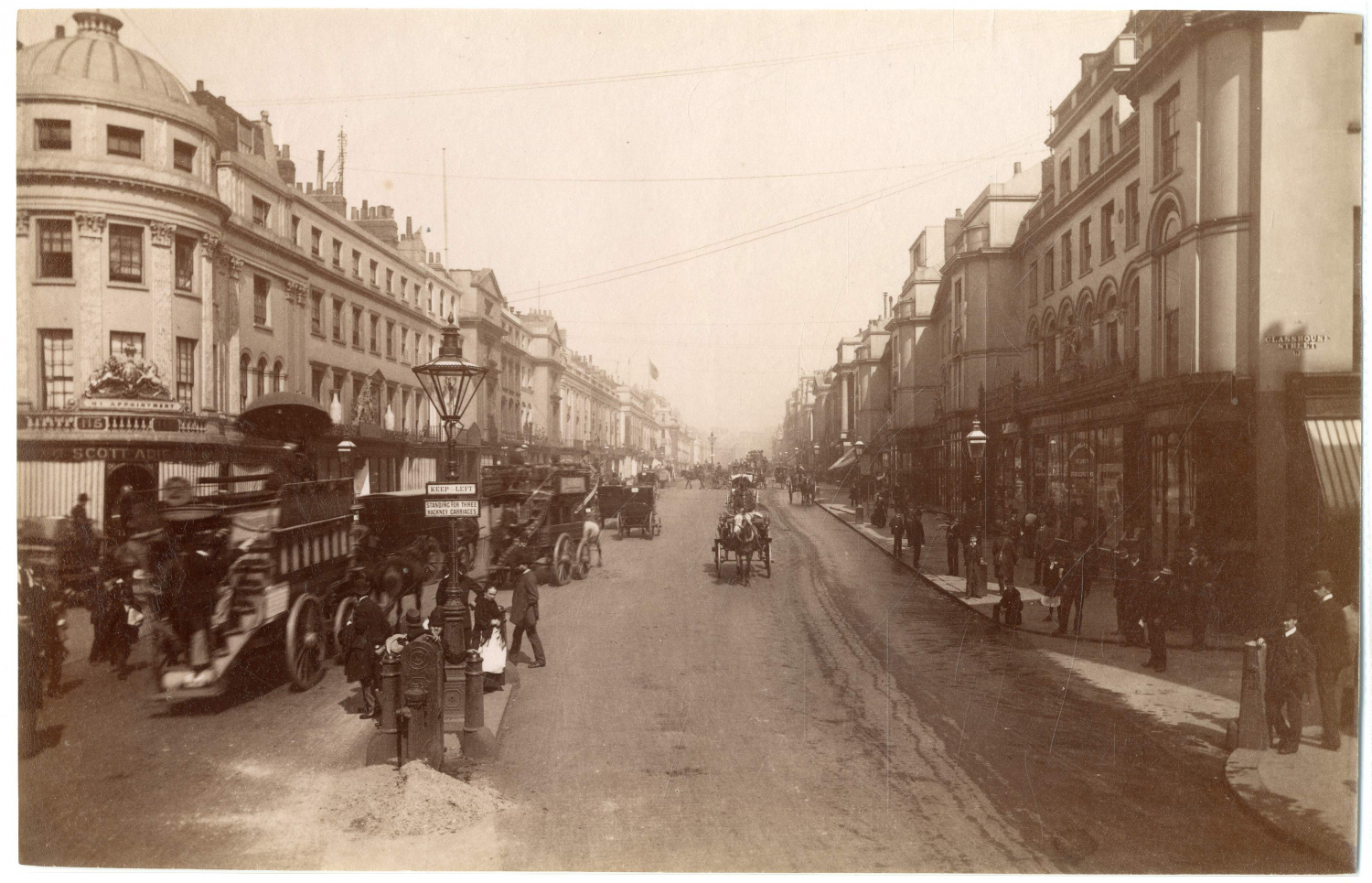The image depicts a bustling city scene captured in an old black-and-white photograph, potentially from the late 1800s to early 1900s. The photo, which has a slight sepia or pinkish tint, offers a perspective looking straight down a wide, central street lined with two- to three-story buildings. The ground floors of these buildings appear to house various businesses, while the upper floors might be used as apartments.

The street is lively with activity; horse-drawn carriages and wagons move up and down, and numerous people, estimated to be in the dozens, stroll the sidewalks on both sides of the street. The men are dressed in plain jackets and bowler hats, common attire for the era. A few specific details stand out: a building with the name "Scott" on it, a man in the background possibly wearing a sombrero, and a dark-colored lamppost near the camera with signs that say "Keep Left" and another unreadable sign below it. The buildings and overall architecture hint at a European style, but the presence of a sombrero suggests it might be somewhere near the U.S. border. The streets appear damp and slightly dusty, indicative of the time period and setting.